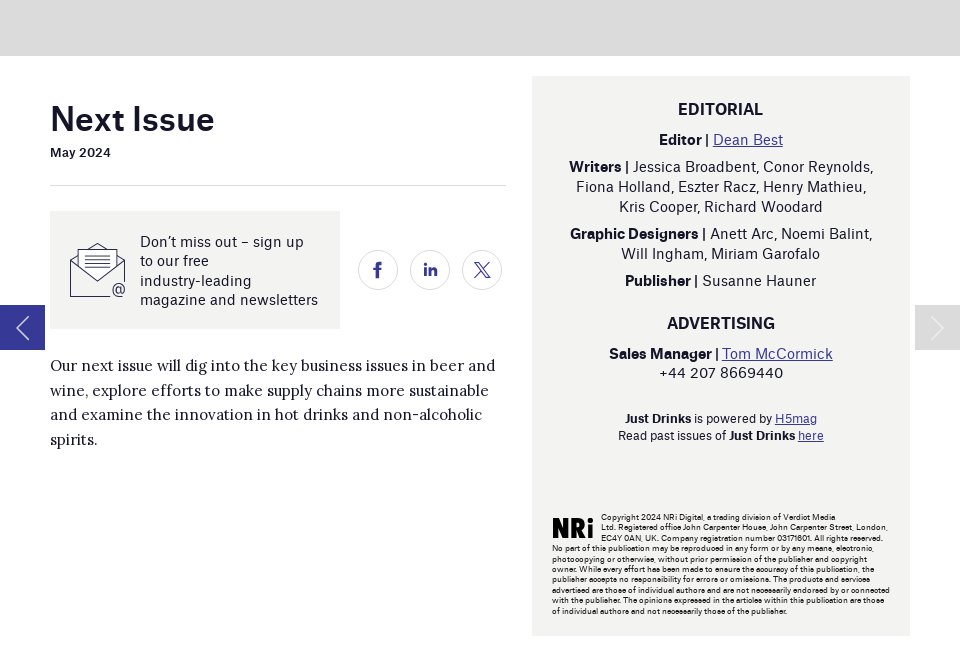At the very top, there's a long gray rectangular box. Below it on the left, the black text reads, "Next issue," followed by the date "May 2024." Another light gray box sits beneath this, containing the message: "Don't miss out — sign up to our free industry-leading magazine and newsletters." 

To the left of this message, an image depicts an envelope with a piece of paper inside. To the right of the envelope, there are three circles: the first with an "F" (likely representing Facebook), the second with "IN" (for LinkedIn), and the third with an "X" (possibly for Twitter). 

Below these icons, the text announces, "Our next issue will dig into the key business issues in beer and wine, explore efforts to make supply chains more sustainable, and examine innovations in hot drinks and non-alcoholic spirits."

To the right, a long gray square features the word "Editorial" in black text at the top. Below, it lists editor Dean Best, with the word "Writers" underlined and followed by the names Jessica Broadbent, Connor Reynolds, Fiona Holland, Estes Rock, Henry Matthew, Chris Cooper, and Richard Woodard. Further down, in black text, it reads "Graphic designers," followed by the word "Publisher." At the bottom, it states "Advertising," with "Sales manager" underneath it in black, and finally, "Tom McCormick" underlined in blue.